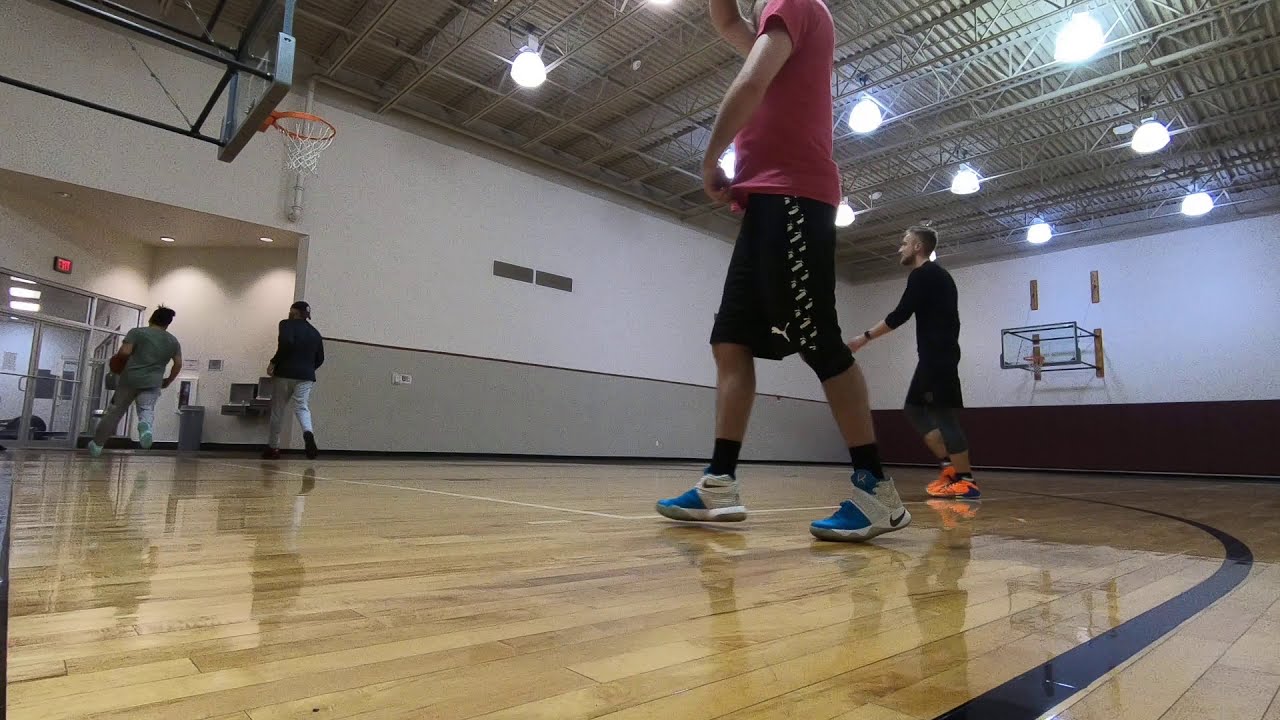This detailed scene captures the bustling interior of a gymnasium during what seems to be a basketball game. There are four individuals on the wooden court, engaged in play. The player closest to the camera is easy to spot, dressed in a red T-shirt, black shorts, and white and blue shoes, dribbling the ball. Right behind him, another player stands out with bright orange shoes, black shorts, and a dark-colored top. Further across the court, one player in a black shirt and white pants, and another in an all-gray outfit, are approaching the active play.

The gym's architecture is notable with its two-tone walls; the longer wall to the side has a white upper section and a light gray lower section, punctuated by two air vents. The shorter wall to the right followed a different scheme with a white top portion and brown lower segment. Two basketball hoops are securely mounted, and above them, the ceiling supports series of large lights, illuminating the scene below.

To the left side of the frame, a set of double doors beneath an exit sign leads to a small hallway lit by overhead white lights. The prominence of the striped painted area, or 'the zone,' marked with a dark blue curved line, is evident on the lower right of the image. Despite the game underway, the vibrant details of the players' attire emphasize the main colors in the scene: white, blue, red, and black.